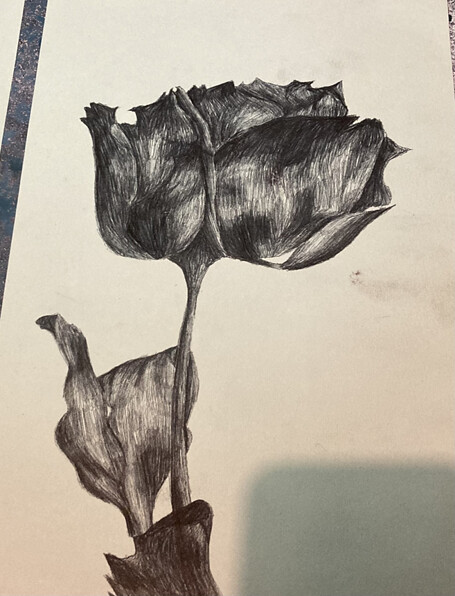The illustration depicts a meticulously rendered side view of a rose, showcasing a high level of detail in its execution. The artist has likely used either pencil, charcoal, or pen, as evidenced by the intricate hatch marks and varying shades of black, gray, and white. The rose is accompanied by clearly defined stems, descending gracefully from the flower. On the bottom left, there is a slightly wrinkled leaf, adding to the naturalistic quality of the drawing. Another area of darker shading on the bottom may represent an additional leaf. The artwork is displayed on a piece of white paper, which casts a rectangular shadow on the bottom right corner. The paper itself rests on a dark, possibly wooden, countertop, which provides a stark contrast to the lighter hues of the illustration.